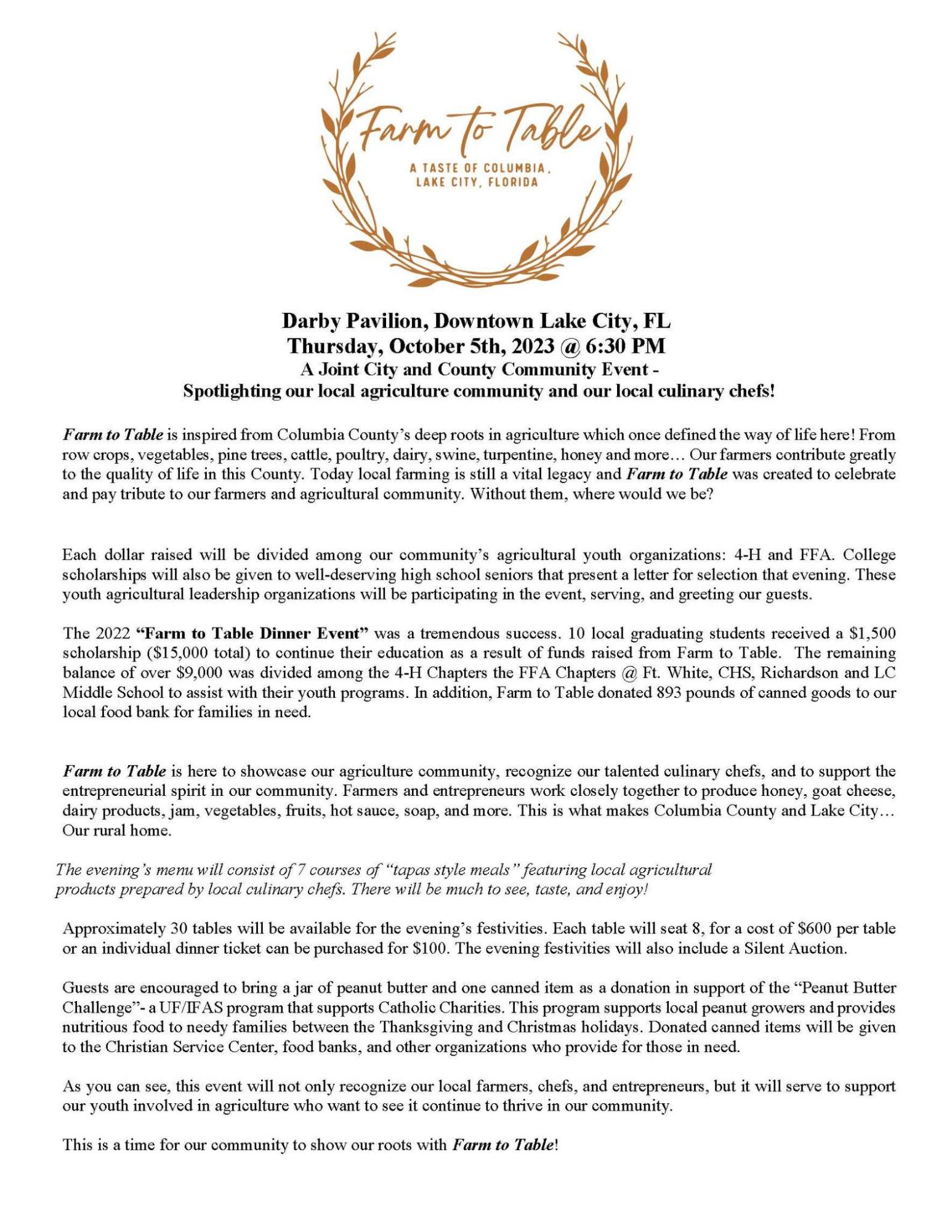This information page highlights an event called Farm to Table, set in Lake City, Florida. At the top, a golden-tan emblem resembling a wreath prominently features the event title "Farm to Table" in a script font. Below, it reads "A Taste of Columbia" with "Lake City, Florida" underneath, all against a white background with bold black text. The event is scheduled for Thursday, October 5th, 2023, at 6:30 p.m. at Darby Pavilion in Downtown Lake City, Florida. This joint city and county community event aims to spotlight the local agricultural community and culinary chefs.

The page elaborates on the importance of the Farm to Table initiative, explaining that it seeks to raise funds for youth agricultural organizations 4-H and FFA. The description mentions that proceeds will support these organizations and generate scholarships for local students, as evidenced by the 2022 event which awarded ten $1,500 scholarships. Attendees can look forward to a seven-course meal prepared by local chefs, along with opportunities to donate. There are approximately 30 tables available, each seating eight people at a cost of $600 per table or $100 per individual ticket. Guests are also encouraged to bring a jar of peanut butter as a donation.